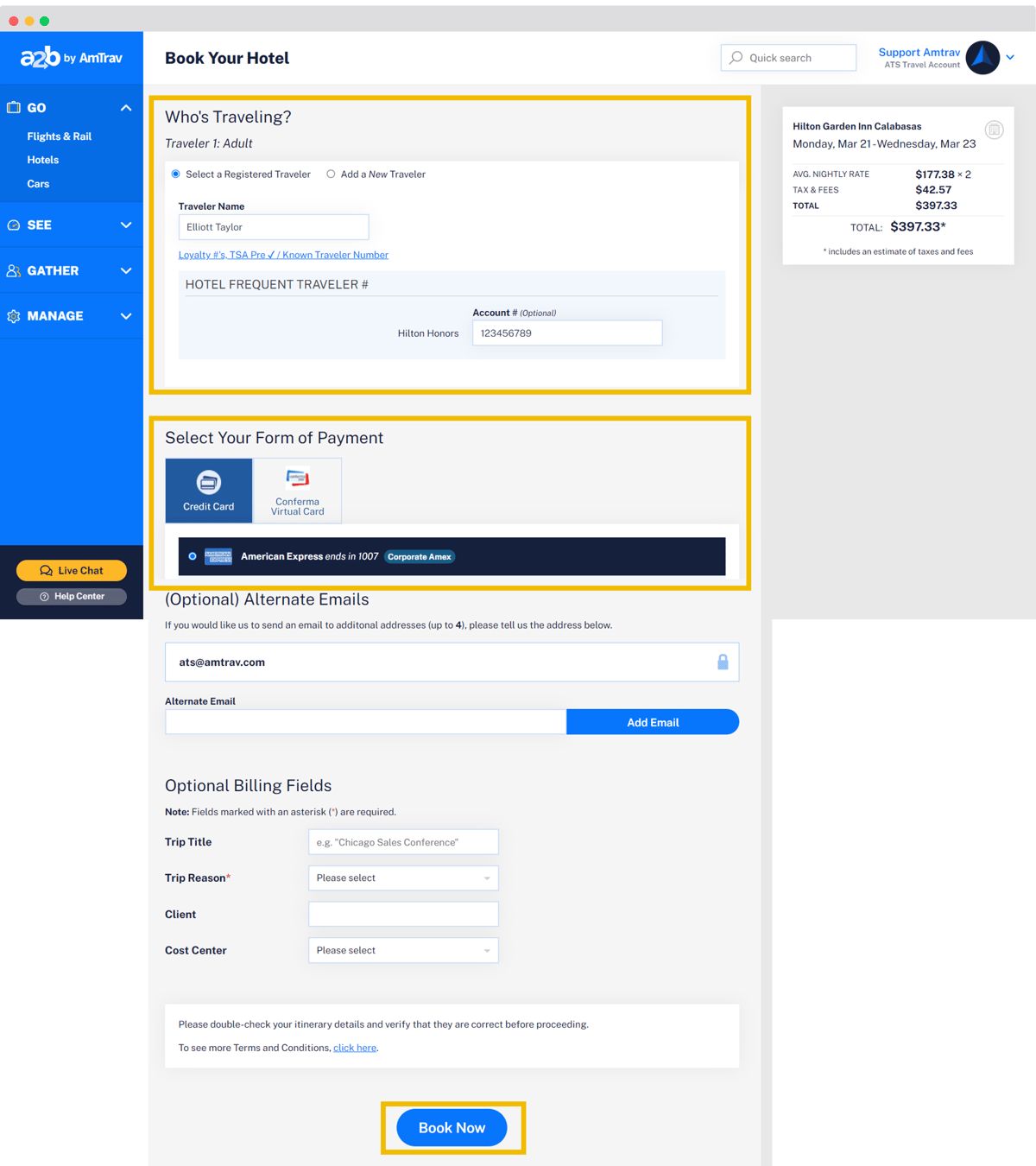The image depicts the interface of a travel booking website called A2B by Amtrav. The main focus is on booking a hotel, with the form displaying fields for traveler information under the section titled "Who's Traveling." The primary details indicate one adult traveler named Elliot Taylor, who is a registered user. His hotel frequent traveler number is associated with Hilton Honors, and there is an input field containing his account number. Additional features of the form include optional fields for alternate emails and billing information. At the bottom, a "Book Now" button is prominently displayed. The payment method selected is American Express, with the projected total cost of the booking noted as $397 on the right side of the interface.